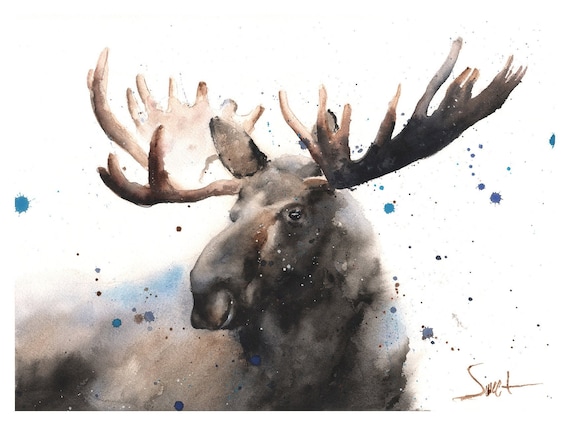This is an oil painting of a moose, predominantly rendered in shades of brown and black, set against a stark black background. The moose's face is the focal point, oriented slightly to the right, showcasing its left eye and left nostril more prominently, while portions of the right eye and nostril are partly obscured. Towering above are the moose’s large, dark brown antlers, adding a majestic touch to its appearance. 

The creature's ears are big and brown like the rest of its body, though the painting blurs out from the neck downward, leaving the full body vaguely defined. Unique to this piece, the moose is interspersed with splashes of blue paint, adding a dynamic contrast to the otherwise earthy palette. These splatters are primarily darkish blue, with a few hints of purple, contributing to an abstract and artistic flair.

A signature graces the bottom of the painting, in light brown cursive, though somewhat illegible. The first letter appears as 'S' and the last as 'T', suggesting a mysterious artist’s mark. Despite the ambiguity of the signature and slight blurriness where the moose's body meets the background, the overall effect is a compelling mix of realism and abstract artistry.